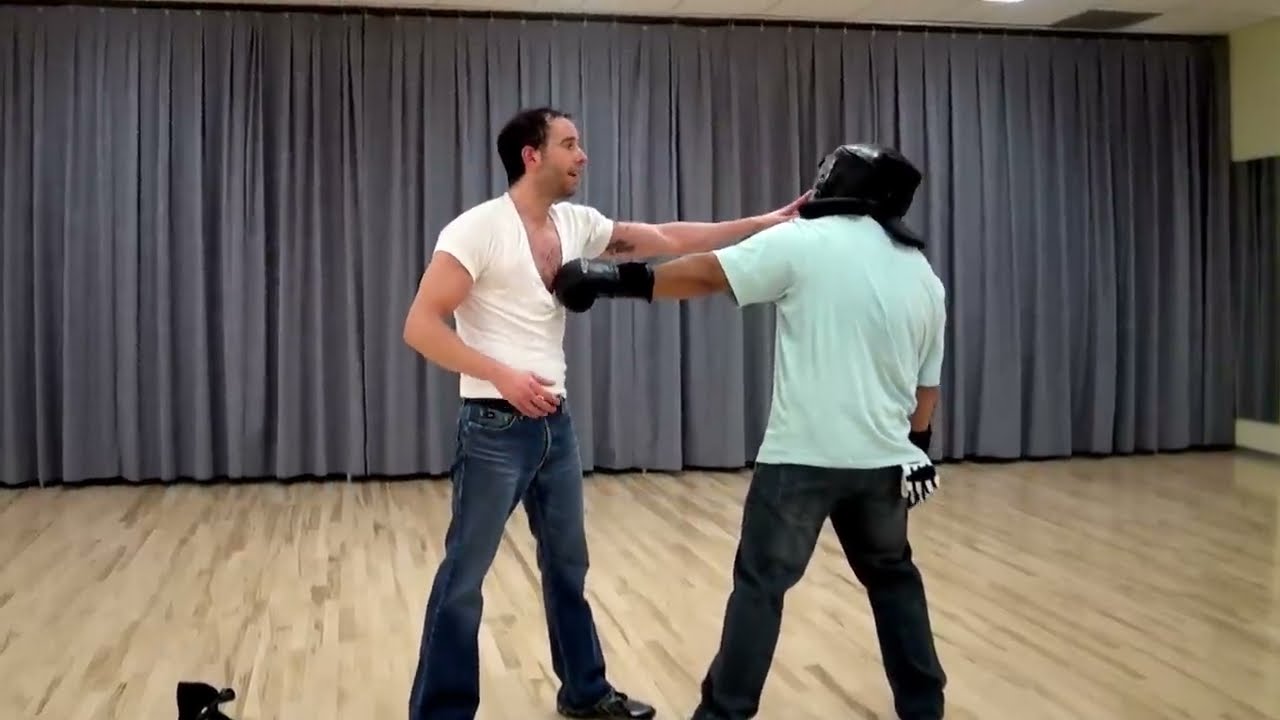In the image, two men are positioned on a wooden stage against a long, heavy gray curtain that runs across the background, suggesting a stage or room divider. The floor of the stage is a sandy blonde color. The man on the left has short black hair and is wearing a white t-shirt, blue jeans, and black sneakers. He is extending his left arm, which is clad in a black boxing glove, toward the chest of the man on the right. His right arm is also extended toward the face of the man on the right, who is wearing a pastel mint-colored t-shirt and dark pants with what seems to be gloves tucked into his back pocket. This man is also wearing black protective headgear that obscures his face. They are engaged in what appears to be a boxing or martial arts practice, with the man on the left adopting an aggressive stance, indicating they are possibly learning or demonstrating fighting techniques. There is an unidentifiable black object on the ground in the foreground on the left side of the image, which might be another glove.